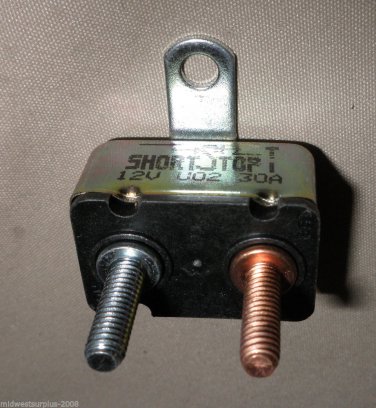The image displays a metal object resembling a combination of a battery and an adapter, screwed into a grainy, textured gray wall that features very tiny light and dark gray speckles. The object is a rectangular silver and black metal box, roughly an inch thick, with a silver flange on top. The flange, which has an arched top and a circular hole in the center, is positioned upside down. Prominently, in black text on the silver side near the top, it reads "Shortstop 12V u02 30A." The main body of the box is horizontally oriented and has a black front plate from which two threaded prongs extend; the left prong is silver, while the right one is copper. Additionally, in the bottom left corner of the black plate, there is barely visible small white text that appears to read "Midwest Surplus - 2008."